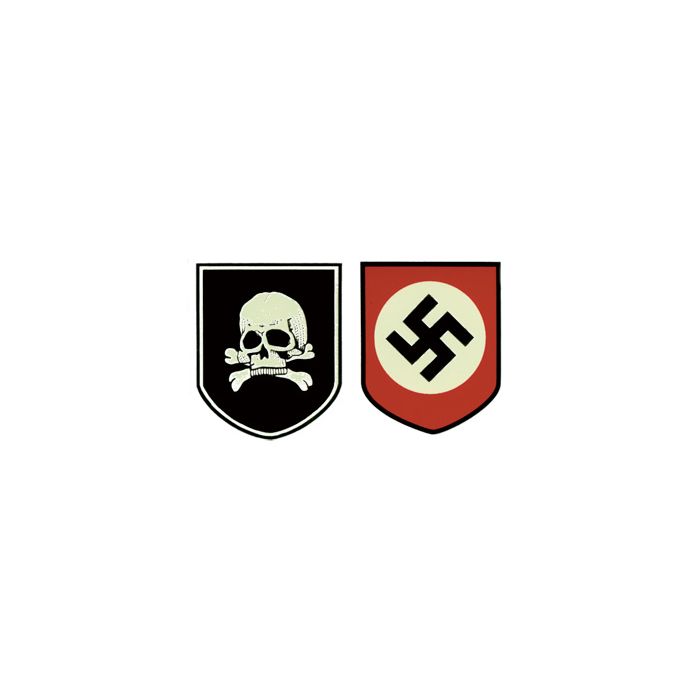The image depicts two digitally recreated patches set against a plain white background. Each patch has three straight sides with a curved bottom forming a point, resembling an arrowhead shape. 

On the left, the patch features a black background bordered by a white band and a thin black line. At its center, there is a prominent white skull with large black eye sockets, and beneath the skull are crossbones.

To the right, the patch has a red background bordered similarly by a black band. In the middle of this red patch is an off-white circle containing a black swastika. Both patches are rendered digitally, emphasizing their simplistic design and stark color contrasts with no additional text or context provided.